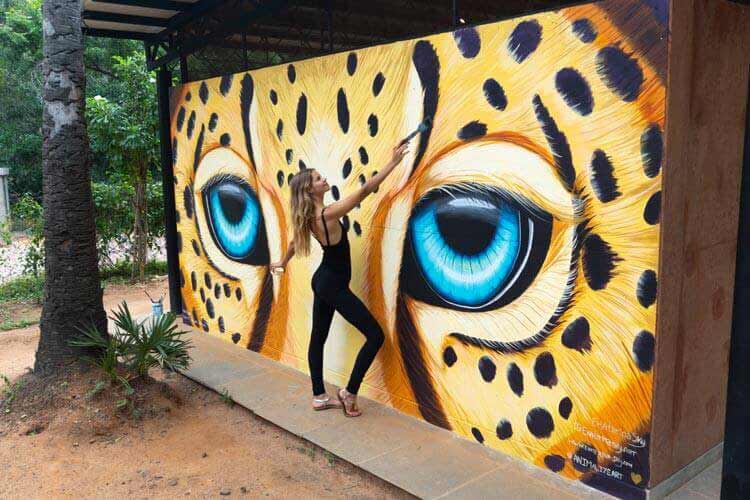The image is a detailed outdoor color photograph taken during the daytime in a forest-like area. The scene captures a young Caucasian woman, approximately 25 years old, with long, slightly wavy, dirty blonde hair parted in the center. She is wearing a black strappy leotard paired with white sandals and long tights. The setting includes vibrant greenery and trees to the left, with a dirt ground or road extending towards the middle and bottom, evoking a jungle atmosphere.

Central to the photograph is a mural on the side of a building, which appears to be a public restroom or a similar facility in a park setting. The mural is an intricate and detailed representation of a cheetah's face, focusing on the eye area and upper nose. The cheetah’s fur is a creamy yellow with black spots, and its striking blue eyes stand out, with whiter coloration around the eyes, contributing to a realistic photographic style.

The young woman is positioned in profile in the center of the mural, holding a paintbrush with her right arm extended above her, seemingly adding finishing touches to the already extensive artwork. Her left arm is extended out to the side. To her left, a small pot filled with paintbrushes sits on a little cement sidewalk platform, though no actual paint supplies are visibly near her. The mural, spanning the side of the building from left to right, has been signed with white paint in the lower right corner, potentially titled "animal heart" or "animal art".